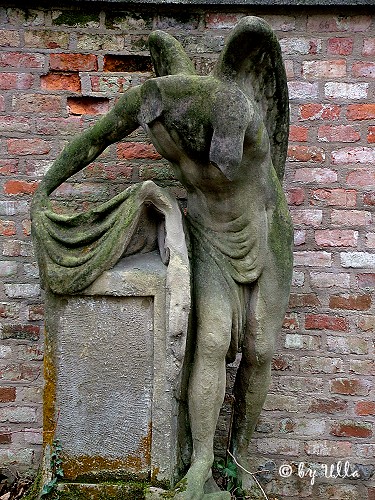This photograph captures an aged, broken statue of a human figure with wings, potentially designed to resemble an angel or mythological character such as Hercules. The statue is notably weathered, with green moss covering much of its surface, highlighting its age. The figure is depicted with a cloth draped around its groin and another piece of carved stone cloth lying next to it on a gray, dirty pedestal. The statue is missing its head and part of its left arm above the elbow, while the right arm extends slightly forward.

The statue is set against a backdrop of partly broken red and white bricks, some of which also bear moss, adding to the deteriorated atmosphere. The winged figure is shown leaning slightly to its left, with the wings rising higher than where its shoulders and head would be. The image is taken during the daytime, illuminating these details clearly. The bottom right corner of the image contains a copyright notice in cursive, possibly reading "Villa" or a similar name. Additionally, a box can be seen near the statue, adding to the sense of disrepair and abandonment that characterizes the scene.